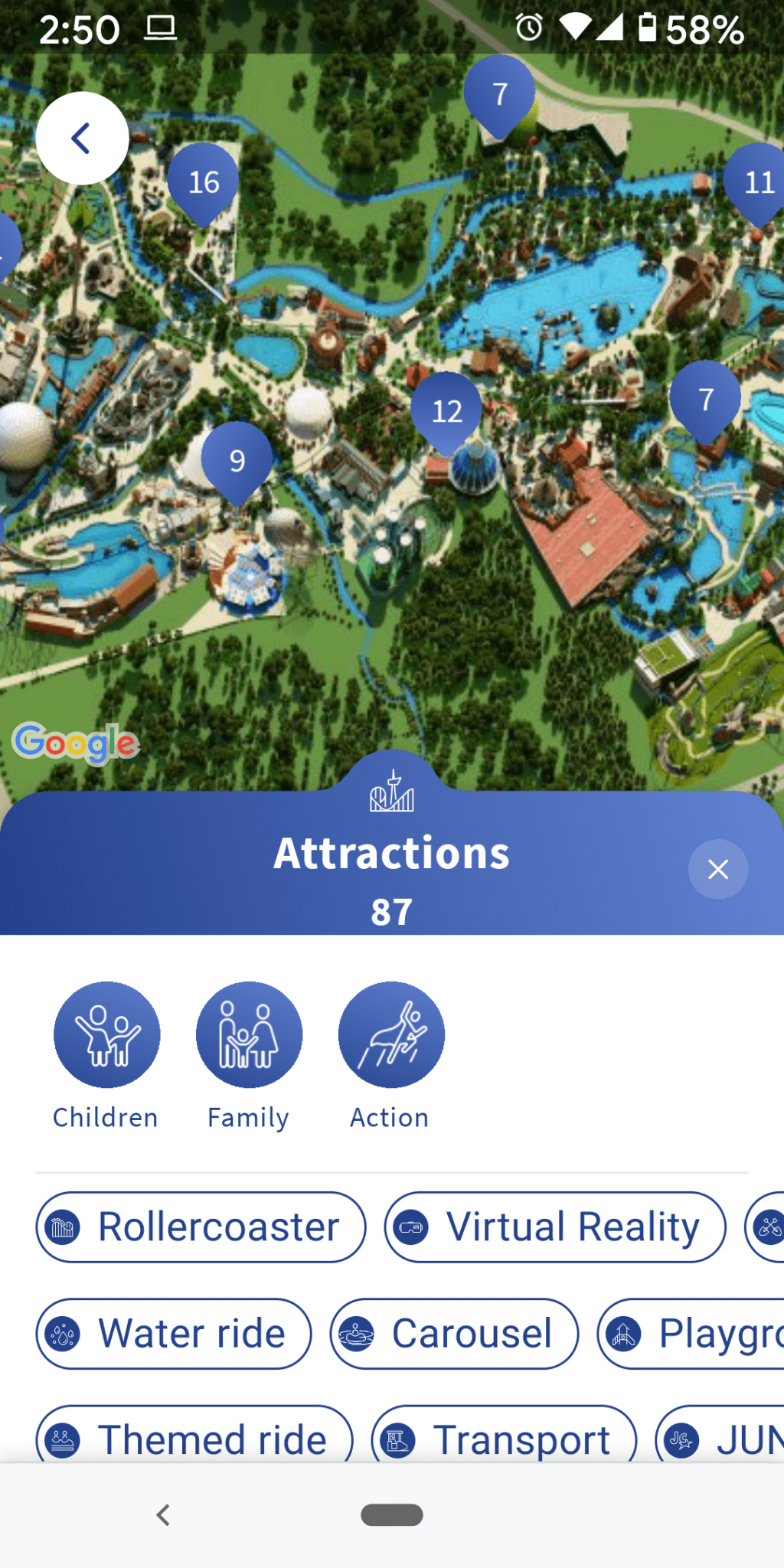This is a detailed screenshot of a meticulously illustrated theme park map. Dominating the top portion of the image, the map features various bodies of water, alongside multiple buildings strategically located between streams and lakes. The landscape is rich with depictions of trees and grass, providing a verdant backdrop to the large buildings scattered throughout.

In the top left corner of the map, there is a prominent white circular back button. Around the map, seven blue map pins are strategically placed, presumably marking key locations within the park. Below the map, a blue banner stretches across the screen, emblazoned with the word "Attractions" in bold white lettering, followed by the number 87, indicating the total number of attractions available.

To the right of the banner, there's an Exit button for easy navigation. Below this section lies a white interface area, featuring three blue circular icons labeled "Children," "Family," and "Action," offering categorized user options. Further down, there is an array of specific attraction categories listed, including "Roller Coaster," "Virtual Reality," "Water Ride," "Carousel," "Playground," "Themed Ride," and "Transport," providing visitors with a detailed overview of the park’s varied activities and ride experiences.